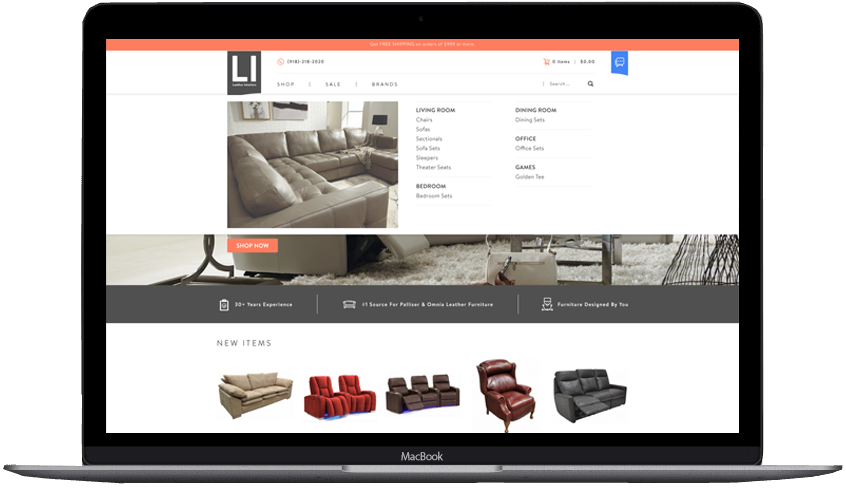A detailed screenshot of a mock-up website is displayed on a MacBook screen, characterized by its distinctive black border and grey bottom edge. At the top of the screen, an orange banner with white, unreadable text is present. Below it is a white section that houses a black rectangle with the letters "L" and "I" in white. This is followed by an image of a grey sectional couch arranged in a three-quarter square formation, set against grey walls. To the right, a living room setup with additional chairs and sofas is visible.

Further down, the website navigation hints at different sections such as "Bedroom," "Dining Room," "Office," and "Games," though the text is blurred. An orange "Shop Now" button is prominently displayed. Beneath this is a narrow grey band, likely the bottom of furniture pieces like sofas or chairs designed for reclining. A grey handbag is placed on a fluffy rug on the floor.

Towards the lower section of the screen, an unreadable grey band with white text is present, even when magnified. Below this, a "New Items" section showcases five images of different couches and chairs. From left to right, there are two red recliners side by side, three dark brown recliners, a single red leather chair, and finally, a three-seater black couch on the far right.